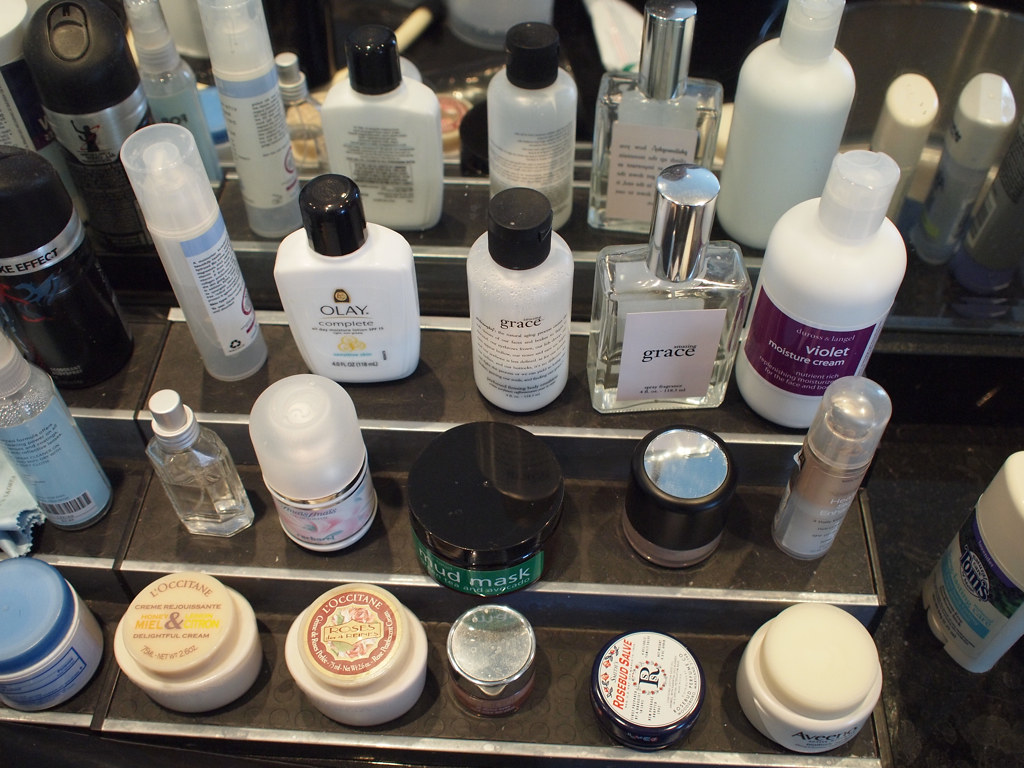The photograph showcases an array of skincare supplies meticulously arranged on a tiered black shelving unit, which has a silver border on the front of each shelf. Viewed from above, the black countertop beneath provides a stark contrast, highlighting the organized display.

On the top tier, from left to right:
1. A can of Axe deodorant spray.
2. A tall, white cylindrical bottle with a clear cap, a brand is unidentifiable.
3. A shorter white bottle with a black cap labeled "Olay Complete."
4. A thin, short, clear bottle with a black cap labeled "Grace."
5. A glass perfume bottle with a silver cap and a pink label that reads "Grace."
6. A taller, wider bottle labeled "Violet Moisture Cream" in a white bottle with a white cap.

Behind these items, a mirror reflects the back of the arrangement, adding depth to the composition.

Descending to the middle tier:
1. A black circular container with a green label that reads "Mud Mask."
2. A clear perfume bottle on the left-hand side without a label.
3. Three additional containers of makeup and creams with unidentifiable labels.

On the bottom tier, dominated by moisturizer-type products:
1. A container labeled "Rosebud Salve."
2. A product from "Aveeno."
3. A container marked "Rose's L'Occitane."
4. A container with the label "Delightful Cream."

Starting a second set of shelves, partially visible at the bottom right of the image, holds an additional item per shelf before being cut off in the photograph.

This carefully arranged set-up effectively highlights the variety of skincare and beauty products available, providing a visually appealing and organized overview.